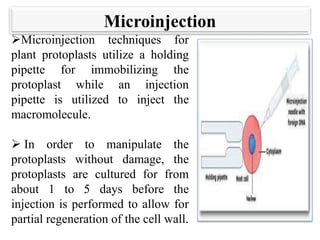The image appears to be an excerpt from a textbook or educational website, focusing on the topic of microinjection. At the top, the title reads "Microinjection." The main content consists of two detailed paragraphs explaining the microinjection techniques used for plant protoplasts. The first paragraph describes how a holding pipette is used to immobilize the protoplast while an injection pipette is utilized to inject the macromolecule into it. The second paragraph explains that to avoid damaging the protoplast during manipulation, the protoplasts are cultured for approximately one to five days to allow for partial regeneration of the cell wall before the injection is performed. To the right of these paragraphs, there is an illustrative diagram demonstrating these techniques. The image shows a needle or syringe approaching a circular object, possibly a protoplast, to visually represent the described injection process. Some accompanying text in the illustration is blurred and not fully readable, but the overall depiction supports the procedural explanation found in the text.